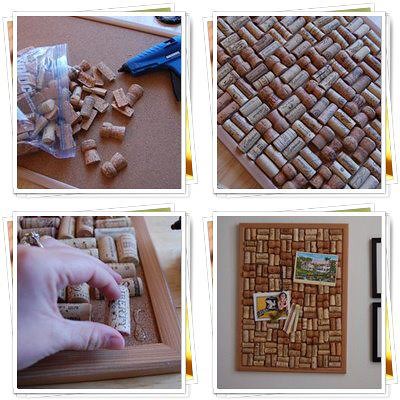This image is a detailed collage of a DIY art project displayed in four color images arranged symmetrically, two on top and two on the bottom, with a white background and a small space between each square image. In the upper left image, there is a cork bulletin board featuring a clear Ziploc bag filled with wine corks that have been split in half, alongside a hot glue gun. The lower left image captures a woman's hand meticulously gluing each cork half onto the bulletin board. The upper right image presents the completed art piece, where the corks are arranged in a visually pleasing pattern. Finally, the lower right image shows the finished cork board hung on a wall, adorned with postcards pinned to it, highlighting its functional and decorative purpose. This collage effectively showcases the step-by-step progression from materials to the finished handcrafted cork board.